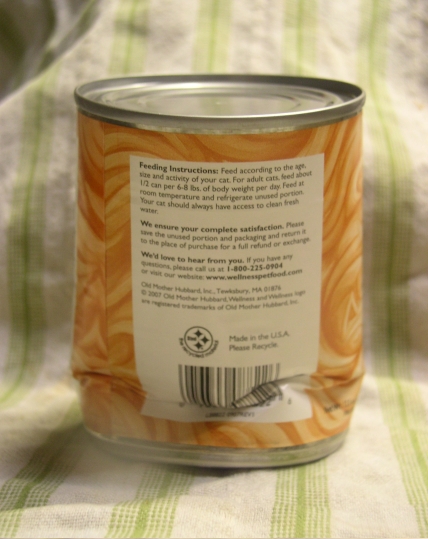This photograph features a dented and partially crushed can of food, positioned on a white pillowcase adorned with green stripes. The can's top is silver and round, typical of a standard food can. The back of the can displays a vertical white section filled with small printed instructions and a barcode at the bottom. The main body of the can is predominantly brown with swirling patterns reminiscent of coffee. The damage to the can is most notable near the bottom, where the crumpling and smashing are more pronounced.